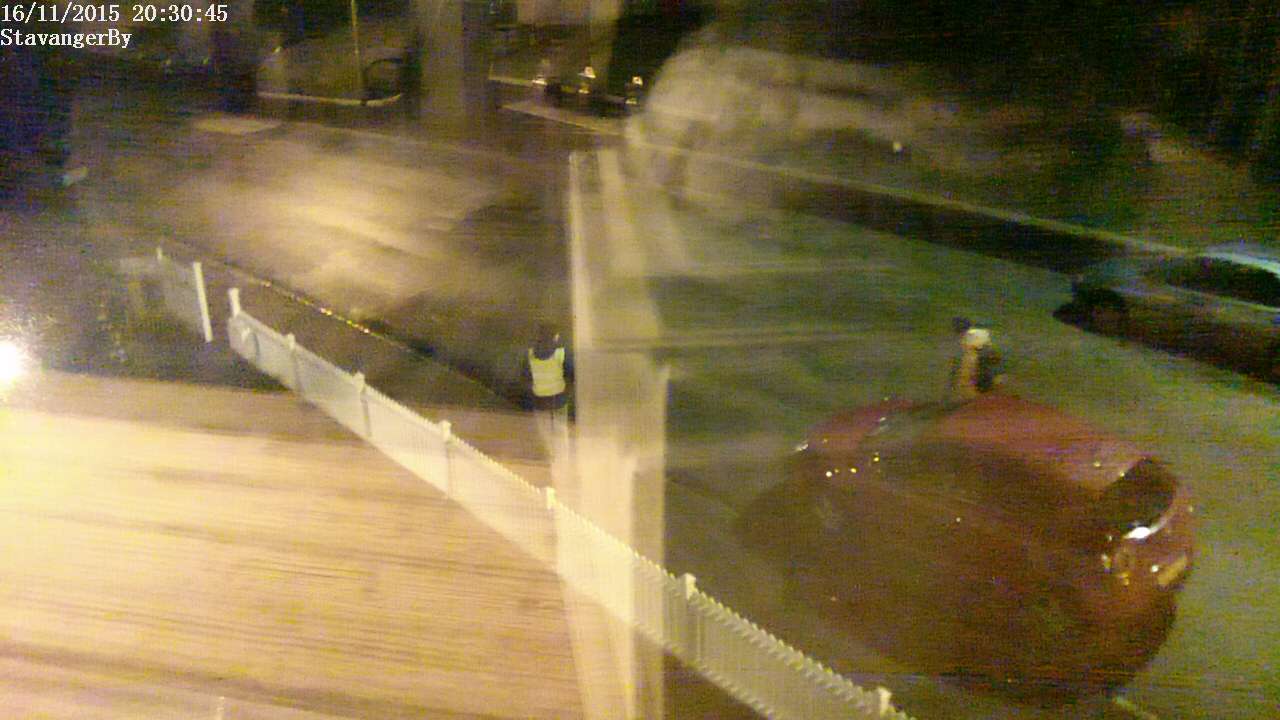This nighttime, color photograph captures a low-light scene that is notably blurry, with reflections or superimposed images adding to its complexity. In the top left corner, white text displays the date "06-11-2015," the time "10-10-45," and illegible writing that appears to say "Sleavon Gelly." The image seems to be taken through a window, adding another layer of distortion. In the lower left corner, a car is visible with two individuals standing in front of it, wearing yellowish high-visibility jackets, suggesting they might be police officers or officials. 

To the left of the car is a white fence, and the car itself appears to be situated on a road. Just above this vehicle, another grey car is visible. This section of the road is bordered by a wall. Towards the top of the photograph, a road junction can be faintly discerned, characterized by a gap in the wall. Another car is approaching this junction at an angle. There is a significant light source that flares up towards the middle left edge of the photo, further contributing to the photograph’s overall blur and obscurity.